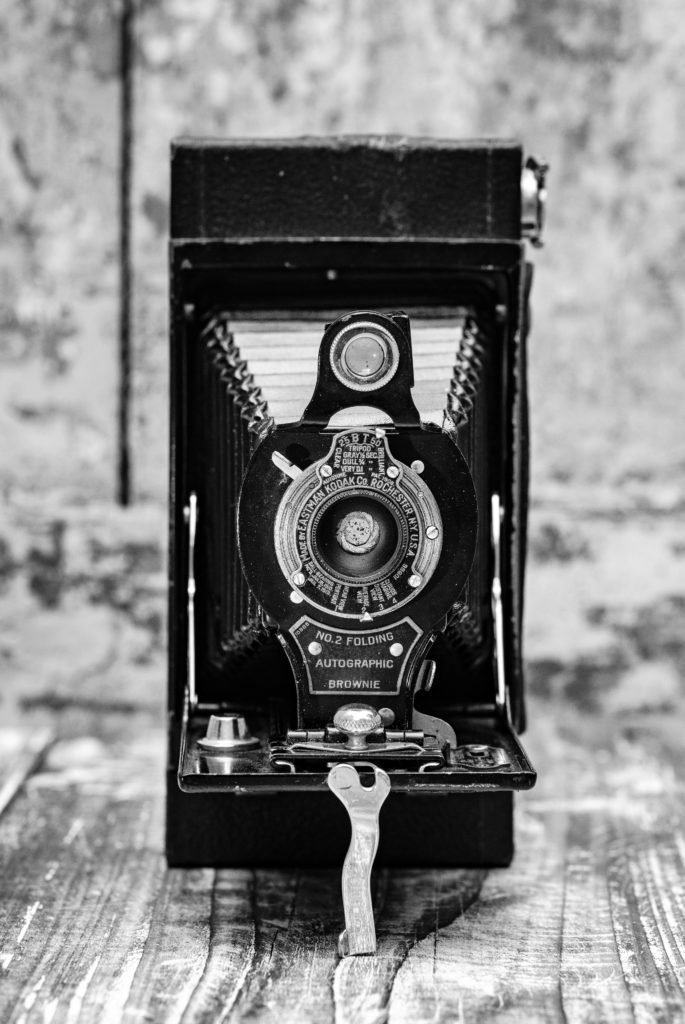This old black and white photograph captures a vintage, rectangular camera, prominently featuring ornate and metallic details that give it a distinctive, antique feel. The camera, identified as a "Number 2 Folding Autographic Brownie," rests on a wooden surface marked by pronounced grain patterns. The foreground prominently showcases a small plaque with the camera’s name, bolted with two silver fittings. In the center of the camera, there’s a circular silver plate which reads "Eastman Kodak, Rochester, New York, USA," surrounding the lens. Above this label is the camera's lens, which is encased in a distinct metal trim. Additionally, a peculiar wrench-like tool is leaning against the camera, suggesting it may be used to adjust its settings. The background appears to be blurred, featuring subtle gray tones that could possibly be bricks, adding depth to the image while keeping the camera as the focal point.